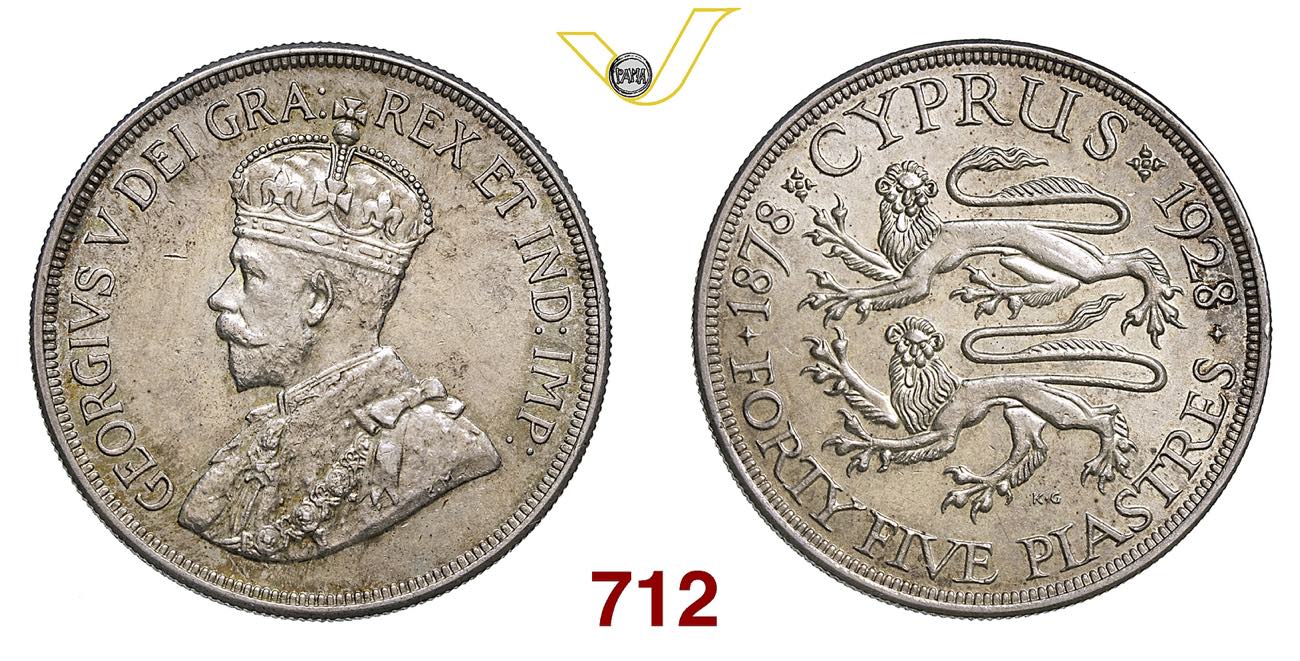The image features both the obverse and reverse sides of a historical coin, with the obverse on the left showing a bearded man wearing a crown, identified as George V. Around his portrait, the inscription reads "GEORGIVS V DEI GRA REX ET IND IMP," which translates to "George V, by the grace of God, King and Emperor of India." The reverse side of the coin, on the right, depicts two mythical lion-like creatures with long tails and talons. The inscriptions on this side include "CYPRUS" at the top, "45 PIASTRIS" at the bottom, and the years "1878" and "1928" on the left and right, respectively. Positioned between the two coins at the top is a yellow-outlined ribbon or logo featuring a small coin, and below it, in red, the number "712."